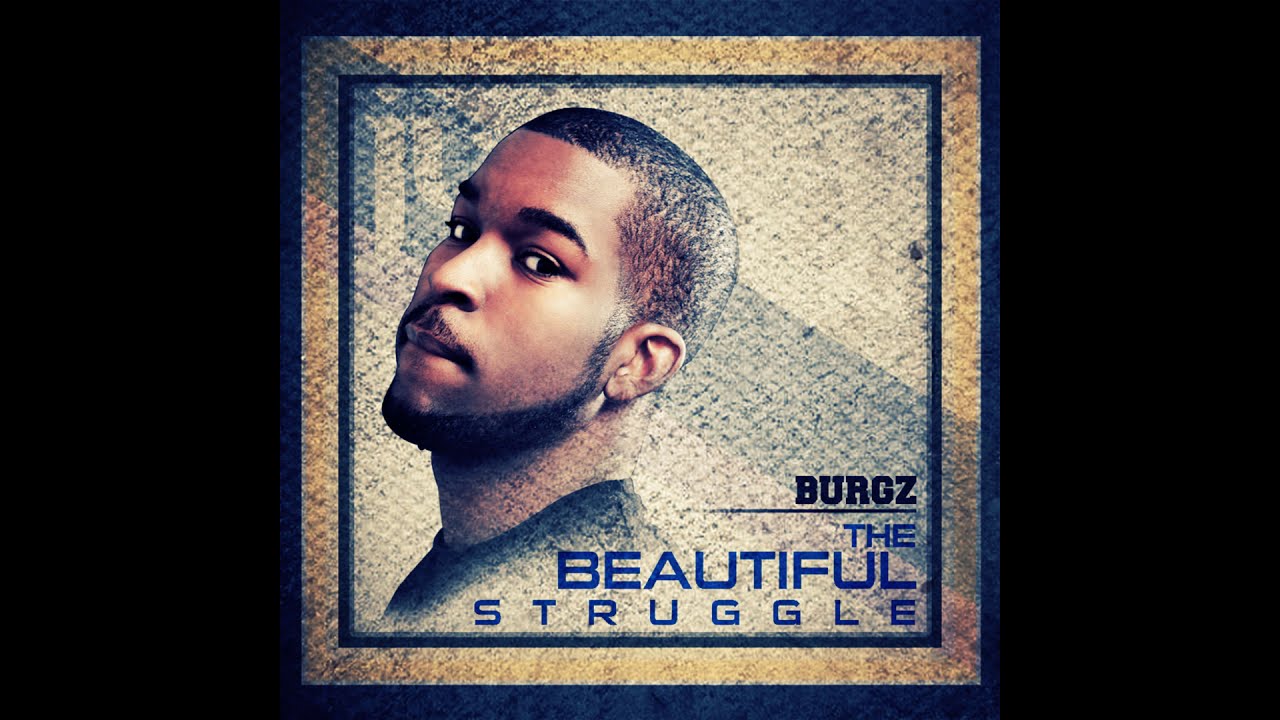The image depicts a digital album cover against a black background, resembling the size of a postage stamp. The cover features a dark-skinned man in profile, identified as "BURGZ" in bold black letters at the bottom right corner. He has closely-cropped black hair, dark eyebrows, a thin mustache, and a trimmed beard lining his jaw. He wears a dark blue shirt, sketch-like in appearance, adding to the artistic quality of the image.

The background of the cover is layered with a dark blue outer frame and a beige inner frame, both detailed with a diamond-dimpled pattern. The man’s head is slightly tilted upwards with his gaze directed to the far left, giving a contemplative vibe. The title of the album, “The Beautiful Struggle,” is prominently displayed beneath his name in a combination of black and dark blue text, stretching from the center to the right of the image. The overall composition of the cover, combining graphical elements and a detailed portrayal of the artist, emphasizes the introspective and expressive nature of the album.